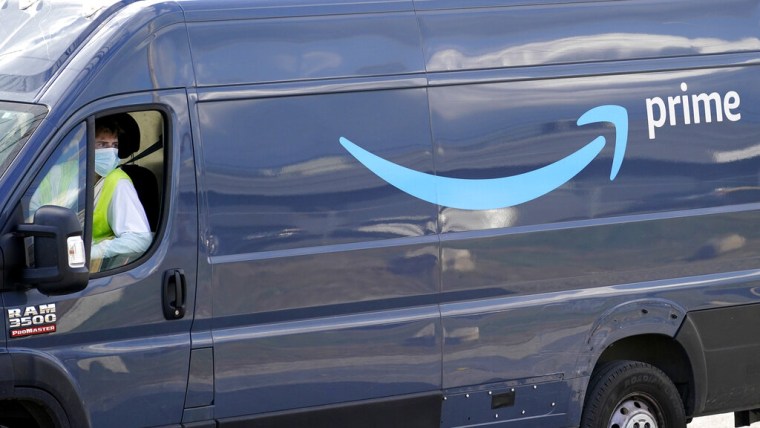This photograph captures an Amazon Prime delivery van, easily identifiable by the prominent Prime logo and the signature Amazon smile logo emblazoned in the middle. The van is a blue-colored Ram 3500, a model commonly used for Amazon deliveries. The scene appears to be taken during the daytime, with natural daylight illuminating both the vehicle and its surroundings. Reflections of a nearby house can be seen on the shiny surface of the van, suggesting recent delivery activity. 

Inside the van, a male driver can be seen. He is wearing a light blue mask, a green vest, and a long-sleeved white shirt. The driver is looking to the right of the frame, possibly checking an address or conversing with someone outside the vehicle. The overall image conveys a typical moment in the daily operations of Amazon's extensive delivery network.